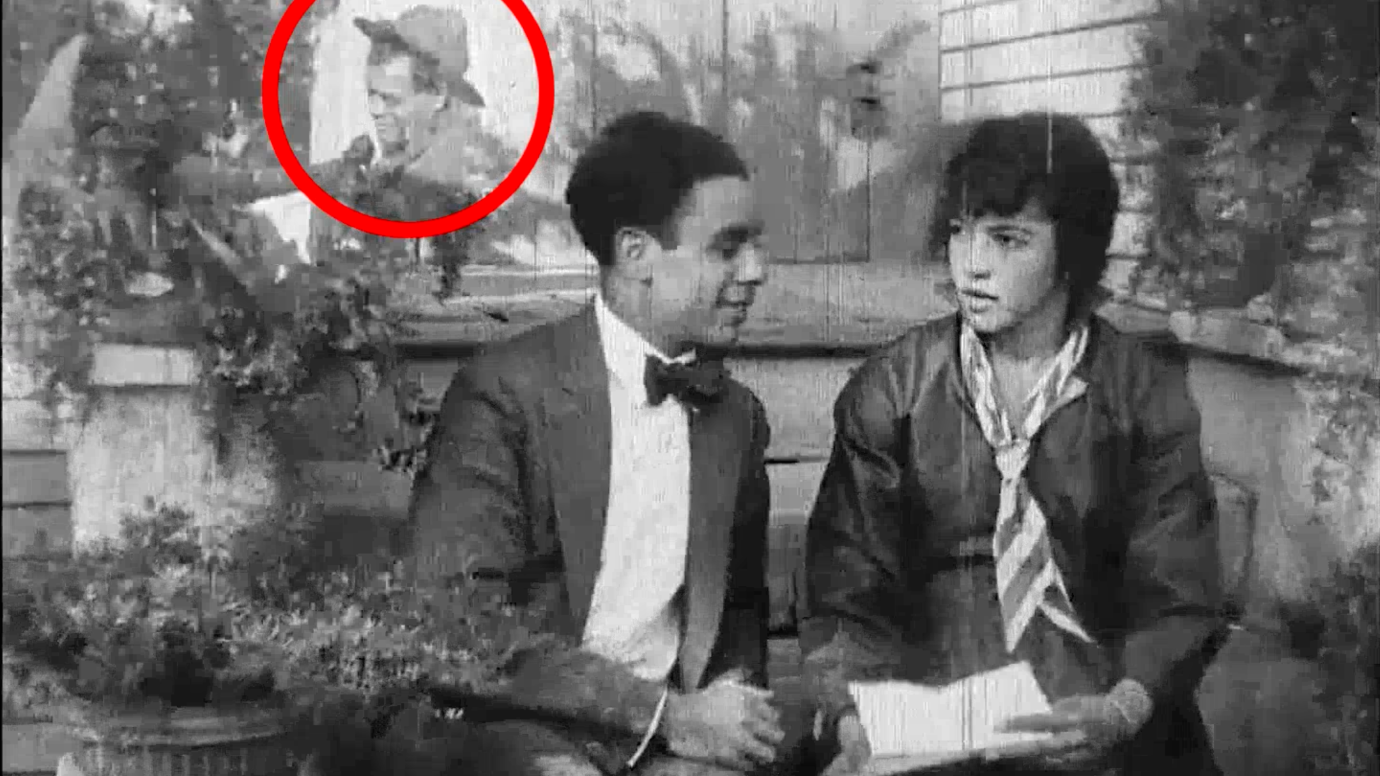This old black-and-white image, possibly a photograph, painting, or digitized artwork, features a young man and woman sitting on a bench in the foreground. The man on the left, of Hispanic or African descent, has black curly hair and wears a suit jacket, white button-down shirt, and a black bow tie. He leans slightly to his left, smiling intently at the young woman beside him. The woman, possibly of Hispanic or Native American descent, with short black hair, dons a dark blouse or dress with a loosely knotted striped scarf around her neck. She holds an open book or piece of paper in her lap and gazes to her right, towards the young man.

Both individuals are seated in what appears to be a garden setting, indicated by potted plants next to the bench and a stone wall covered in ivy in the background. Prominently behind them is a mural on the stone wall, depicting a man with a hat, a mustache, and a goatee, hinting at the early 20th century or late 19th century style. This man's head and shoulders are highlighted with a red circular arrow, drawing attention to his presence in the image. There is no visible text or horizon, and the focus remains on the interaction between the two seated individuals and the mural behind them. This engaging scene could originate from a still frame of an old movie or simply depict a nostalgic moment captured in vintage style.